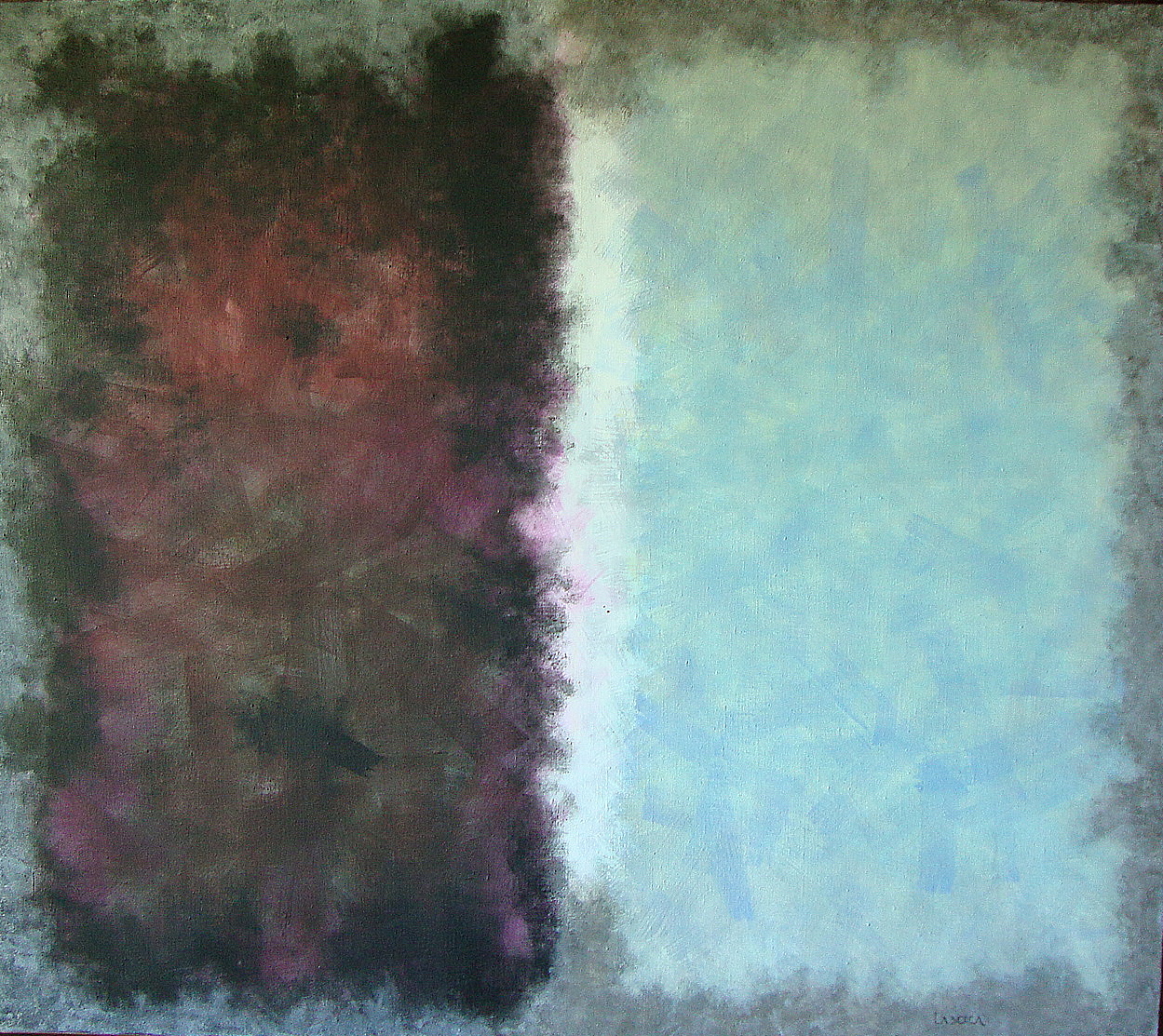This slightly wide rectangular painting is framed by an uneven, grayish-blue border that fades at the edges. Dominating the left half of the artwork is a vertical, uneven rectangular shape, starting with a black base that transitions into layers of brown, purple, and increasingly red hues towards the top. On the right half, a tall rectangular form is filled with varying shades of blue, including sky blue, intermingled with thin streaks of white paint. Separating these two rectangles is a thick white line that seamlessly blends their edges together. The textured brush strokes are visible throughout the piece. In the bottom right corner of the border, there is a small, barely legible name that appears to spell out "L-A-S-C-A."